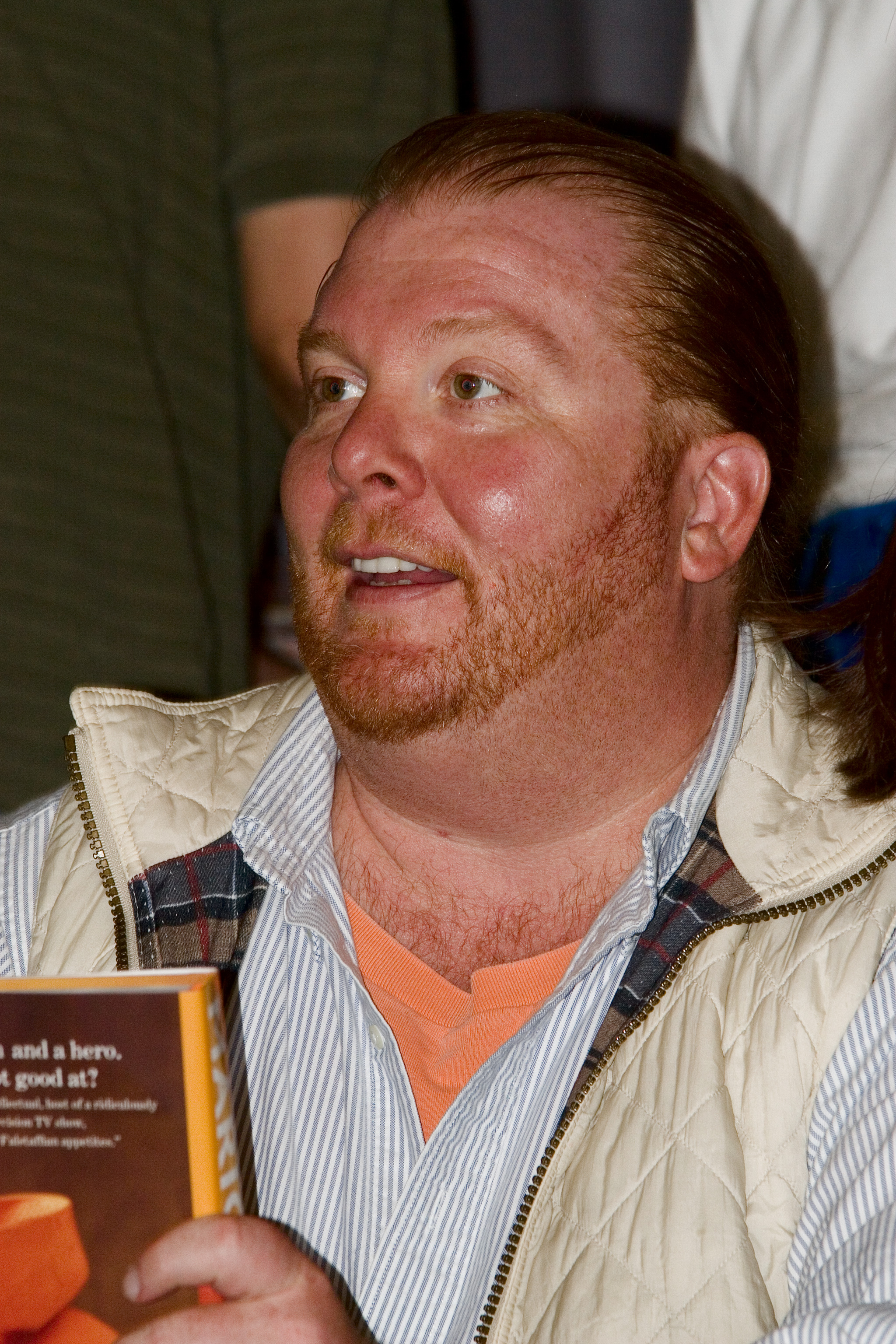In this detailed image, we see chef Mario Batali seated and facing the left side of the frame, smiling faintly. His distinct slicked-back red hair cascades past his shoulders, and he sports a neatly trimmed, clean-shaven beard and mustache. Dressed in a peach-colored V-neck shirt peeking out beneath a white and blue pinstripe collared shirt, Mario adds a layer of sophistication with an off-white vest that is unzipped, revealing a subtle checkered pattern of brown, blue, and red on its inner lining.

In his left hand, visible in the lower left corner of the image, he holds a hardcover book with a yellow binding and white lettering. The back cover of the book, which is brown with orange accents, prominently displays the partially visible words "end a hero good." Two other people are seen standing behind him, suggesting that the setting might be a book signing or reading event. The image captures Mario from the chest up, detailing his attire and the intriguing elements of the scene around him.